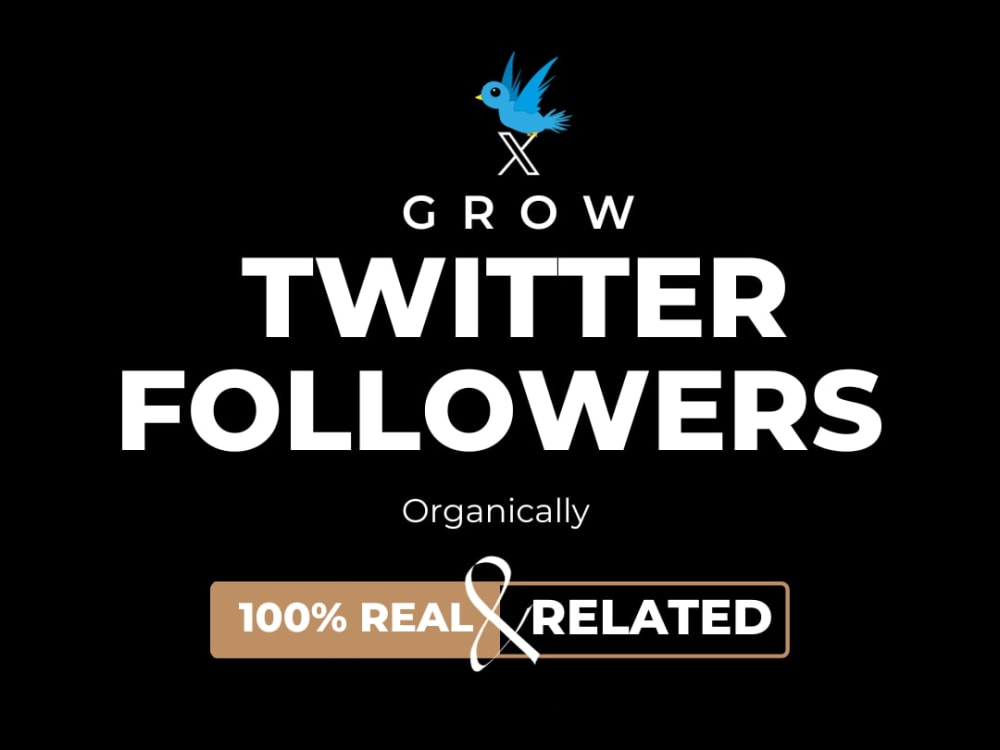The image features a pitch-black background, creating a stark contrast that accentuates its foreground elements. At the top of the image is a small blue bird, characteristic of Twitter, with its wings raised as if in the midst of landing. The bird has an orange-yellow beak and black eyes, and it is positioned directly on top of the Twitter X logo. Below the bird, the text "Grow Twitter Followers" is displayed prominently, with "Twitter Followers" in a noticeably larger white font for emphasis. Beneath this, the word "organically" appears in smaller white font.

At the bottom of the image is a rectangular box divided into two halves. The left half is tan-colored with a tan border encasing the entire box, and it features the words "100% Real" in white font. The right half of the box is black, with the word "Related" also in white font. A large ampersand symbol (&) connects the two halves, reinforcing the message that the followers are "100% Real & Related."

Overall, the caption for the image reads: "Grow Twitter Followers organically. 100% Real & Related." The design and text convey a clear and direct message emphasizing organic and authentic growth of Twitter followers.